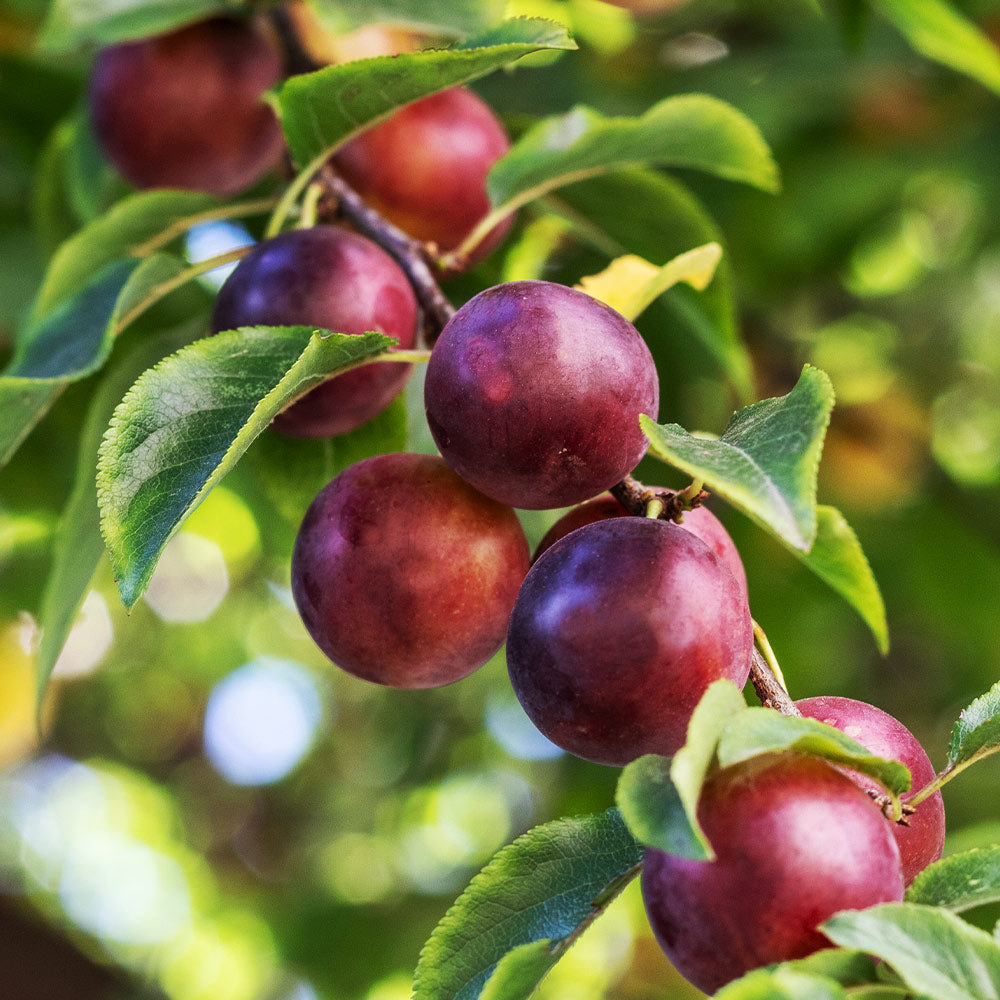This vivid colored photo captures a branch of fruit-bearing plant with approximately six purple-reddish plums prominently displayed in the foreground. These plums vary in shade, with some appearing darker and others brighter, glistening with reflections likely from sunlight. The plums are clustered around a twig connected to a larger tree, adorned with lush green leaves. While the foreground remains sharply in focus, revealing the fine details of the plums and their smooth, reflective surfaces, the background is blurred, showcasing the green foliage and additional plums in a soft focus. This backdrop of greenery hints at a sunlit environment, enhancing the overall natural aesthetic of the image.